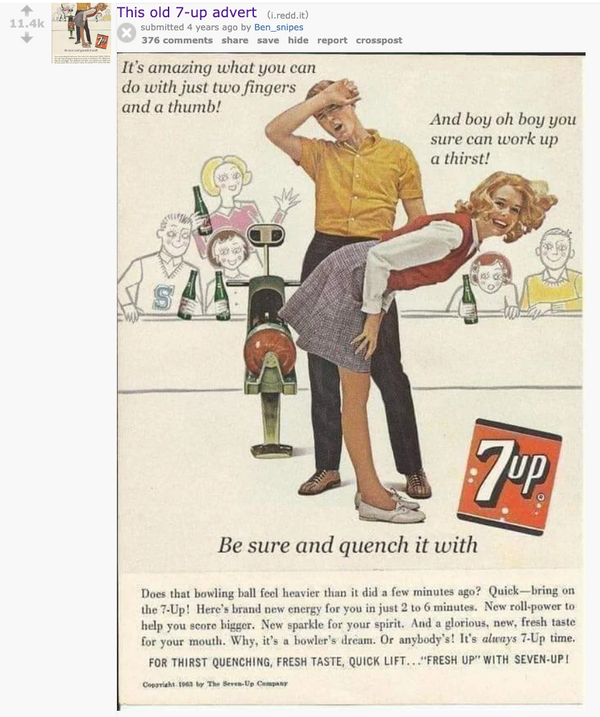The image is a screenshot of a Reddit post featuring a vintage 7-Up advertisement, shared by user ben_snipes. The post has the title, "This old 7-Up advert," which is displayed in purple text indicating it has been clicked on. The Reddit layout is the older white background version, showing the post's upvote count at 11.4K. 

Most of the image is dominated by the ad itself, characterized by its old and slightly pixelated look, reminiscent of the 1950s or 1960s. The ad features a blonde woman in a red cardigan, white blouse, and skirt, bending over in a bowling alley setting. She is depicted in profile view but turns her head to smile at the viewer. Behind her, a man in a mustard-colored shirt and brown pants appears tired, wiping his forehead with the back of his hand. Both figures are surrounded by simple, hand-drawn illustrations of people holding 7-Up bottles. 

Several pieces of text add to the ad's playful, innuendo-filled tone. In the top left, it reads, "It's amazing what you can do with just two fingers and a thumb," while above the woman's head it says, "And boy, oh boy, you sure can work up a thirst." At the bottom, large black text states, "Be sure and quench it with 7-Up," next to the vintage 7-Up logo—a red square with "7-Up" in white and a black drop shadow. Below this is a lengthy promotional message extolling the beverage's ability to refresh, energize, and increase bowling performance in just a few minutes, concluding with, "It's always 7-Up time. For thirst quenching fresh taste, quick lift, fresh up with 7-Up."